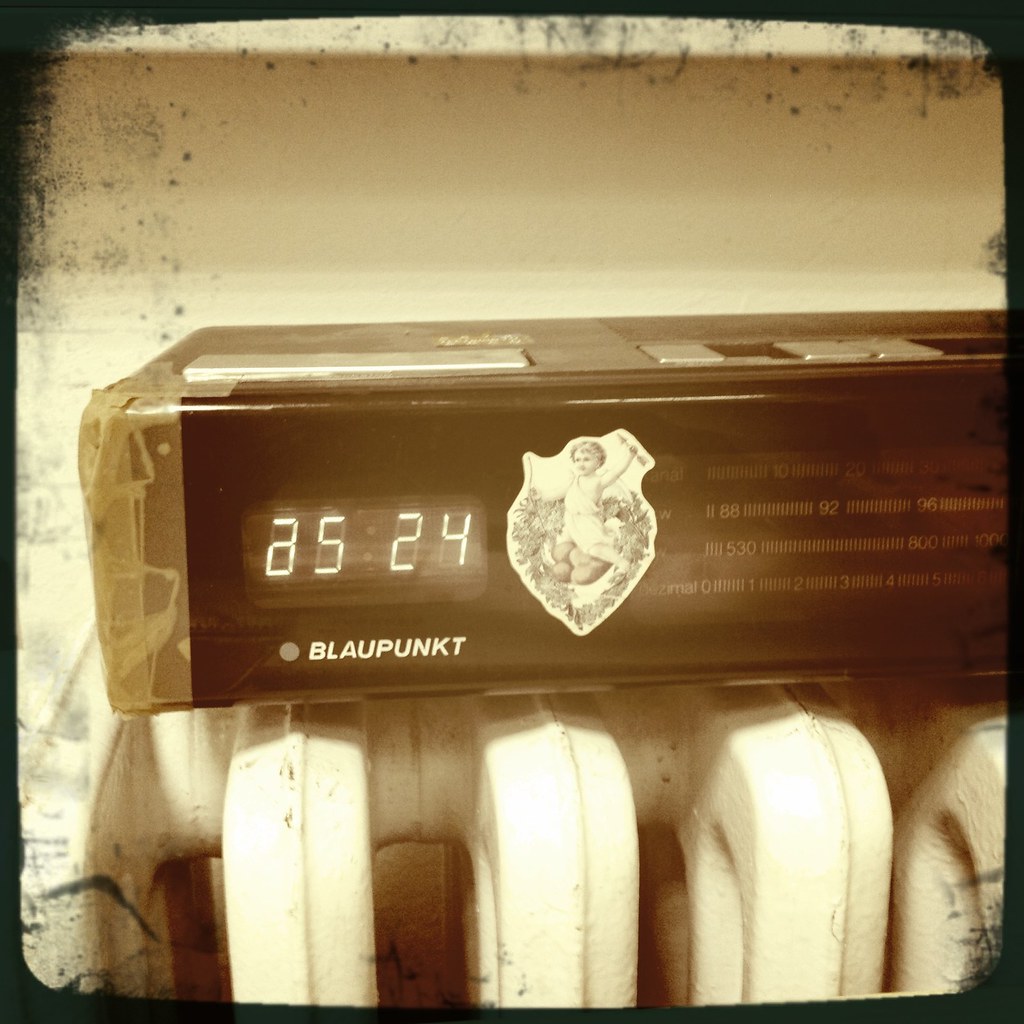This photograph captures a vintage-style, radiator heater, prominently positioned at the center. Rendered in black-and-white with a distinctive sepia tone, the image exudes an antique quality. The photograph appears to have undergone a traditional film development process, resulting in visible artifacts such as rough edges, scratchy dots, and cracks scattered throughout the image. The corners of the photo are notably faded, enhancing the nostalgic atmosphere. The radiator heater itself, likely white or a light color, contrasts with the sepia filter. Atop the heater rests a rectangular digital display, which modernizes the scene slightly yet still manages to blend into the overall rustic aesthetic. This combination of old and new elements, coupled with the photograph's visibly aged texture, creates a compelling historical ambiance.